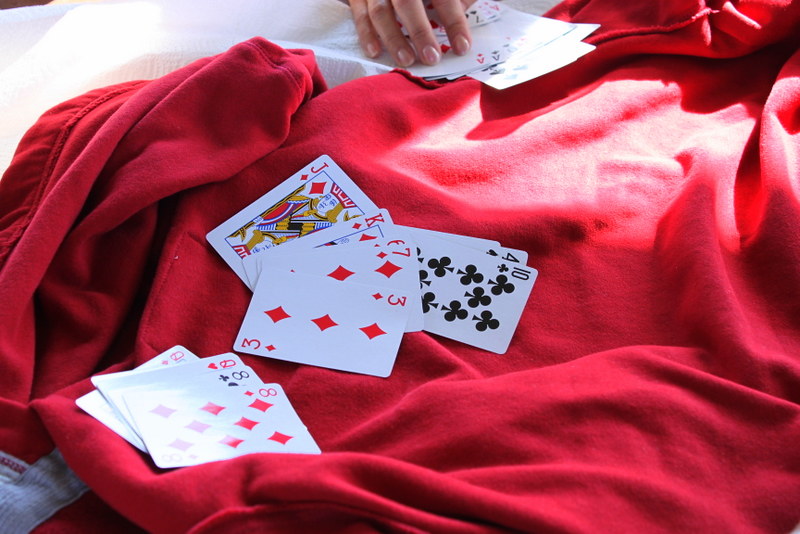This photograph features an arrangement of playing cards spread out on a bed, illuminated by sunlight. In the center, a hand with fingers visible is holding a set of cards, evidently in the process of organizing them into three distinct groups. In total, there are two stacks of cards. The hand is seen organizing cards into groups of three, five, and four. One stack in the foreground is slightly separated from the main group.

The bed is adorned with a red blanket, under which a white sheet can be seen. The cards appear to be grouped in pairs, with two 8s and two queens forming one set, and two aces visible in the other stack. This detailed arrangement suggests a game or an act of sorting the cards based on certain rules. The sunlight streaming in adds a warm glow to the scene, highlighting the intricate layout of the cards and the surrounding textiles.